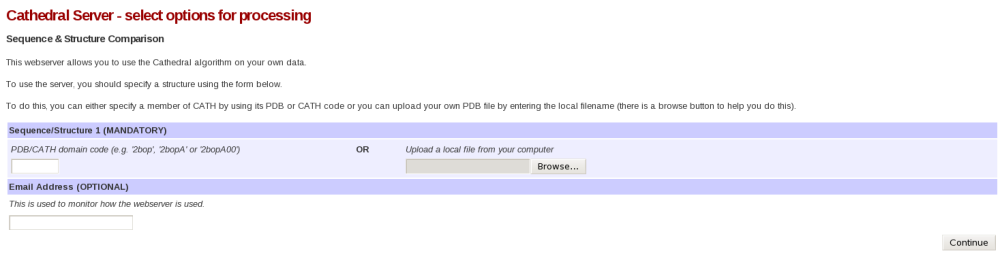**Detailed Description:**

The screenshot features a user interface with a white background and various server selection options highlighted in red. This interface is part of a cathedral server designated for sequence and structure comparison processing. Users can leverage cathedral algorithms to analyze their own data.

The web server provides a form for specifying structures. Users have the option to input a CATH code by either entering a member of CATH (denoted as "C-A-T-H") with its PO-B (Protein Observed By) code or uploading a local PO-B file from their computer. Instructions suggest entering the local town name in parentheses when uploading files. 

A prominent "Browse..." button is available to facilitate file selection. The section labeled "Sequence Structure 1 (Mandatory)" indicates its importance in the process.

The interface includes an email address field, which is optional, purposed for monitoring how the server is utilized during the webinar. Adjacent to the email field is a gray rectangle with the text "Browse…".